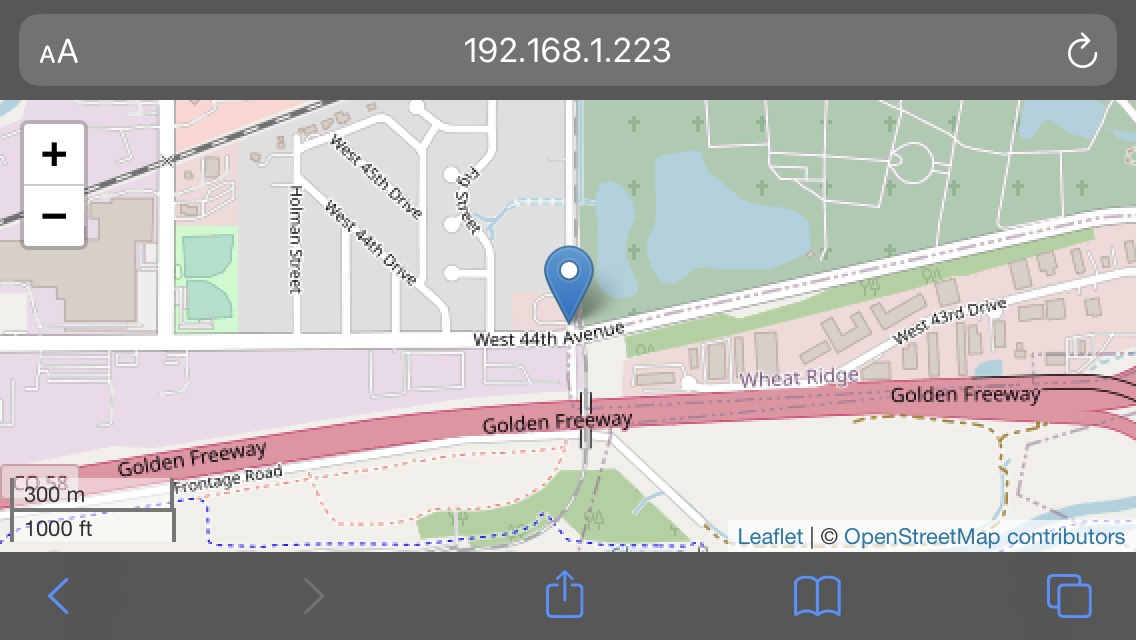The image displays an iOS interface with the IP address "192.168.1.223" prominently shown at the top. On the upper right corner, there is a reload button. On the lower section of the screen, there are several icons: a blue share button on the left, a blue book icon on the right, and two blue overlapping squares further to the right. Position-wise, the bottom left of the image reads "300 meters, 1,000 feet."

The central portion of the screen features a map segment labeling "West 44th Avenue" and "Golden Freeway." On the left side of the map, a neighborhood area is displayed, while the right side includes a garden. The map and interface elements suggest navigation through a specific locale within an iOS mapping application.